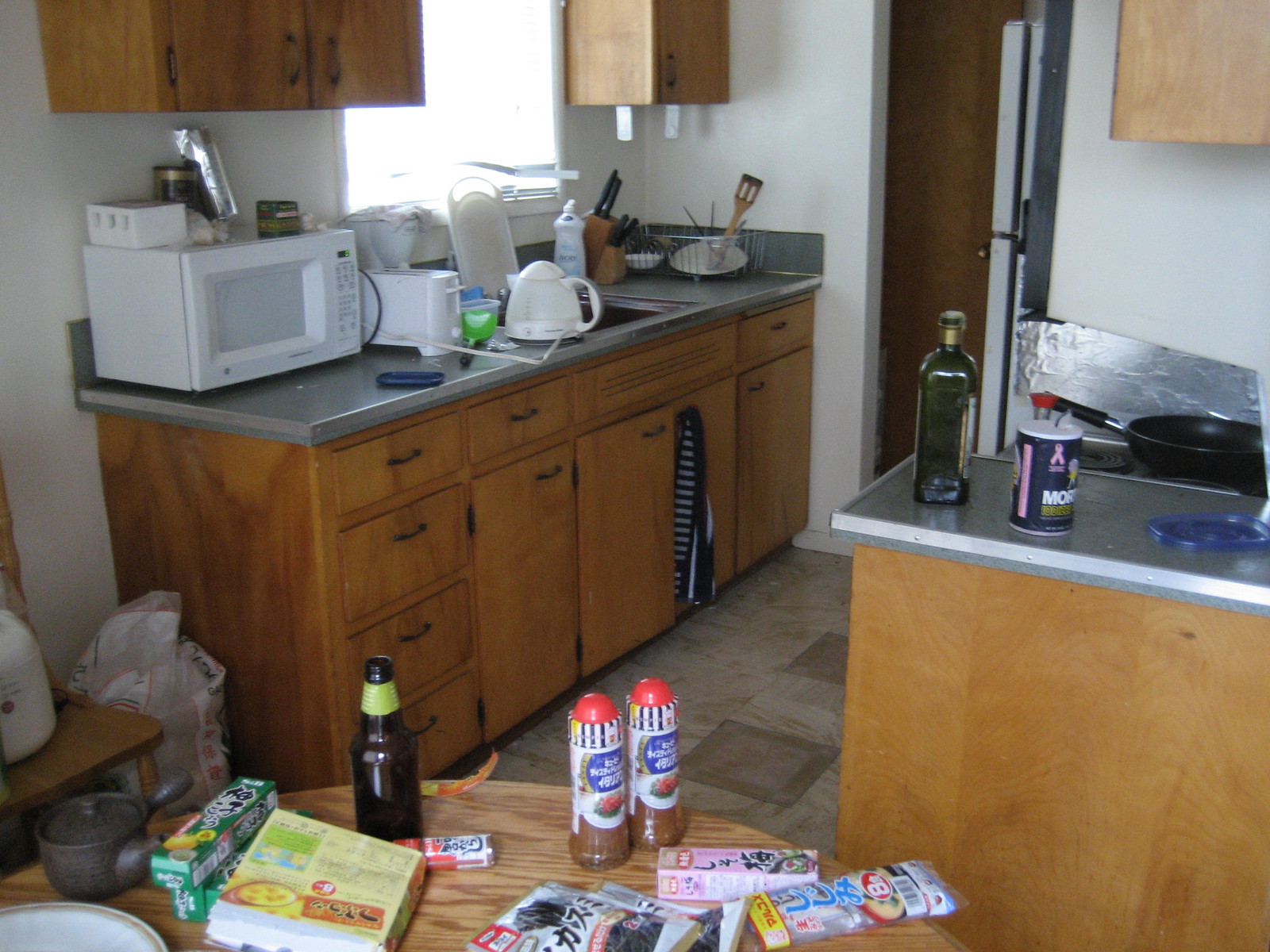**Detailed Caption:**

The image depicts a bustling kitchen scene in color. In the bottom left, partially visible is a wooden chair holding a white item, possibly a gallon of milk or a rice cooker. Across the bottom of the photo, part of a round table is visible, notably featuring a brown ceramic Japanese-style individual teapot, designed for steeping loose leaf tea, accompanied by two small boxes, similar to those used for packaging prepared wasabi. Also on the table lies a cookbook, face down, and a brown glass bottle, which resembles a beer bottle. Scattered around the table are food packets commonly used for nori or broth, along with a long box likely containing a tube or bottle. Two identical bottles with red tops, potentially seasoning shakers, stand upright. 

Towards the upper part of the image, a kitchen counter spans the photo, cluttered with various items such as a white microwave, a two-slice toaster, a suspected electric tea kettle, cutting boards, colanders, a knife block, utensil caddies, and dish soap. The countertop, a gray hue, lies atop medium-colored wooden base cabinets which feature several drawers and doors. Above the counter, there are wall cabinets flanking a large window emitting bright daylight, creating a somewhat blinding effect.

From the right wall cabinet hang two empty under-cabinet paper towel holders. To the right, another room is accessible through a door. Additional cabinetry and an electric coil stovetop occupy the right side of the image, with a frying pan resting on the cooktop. The counter bears another bottle, possibly olive oil, and a recognizable Morton salt container, identifiable by its breast cancer awareness red ribbon logo and pink stripe. The kitchen floor is covered in linoleum, patterned with tan and brown squares.